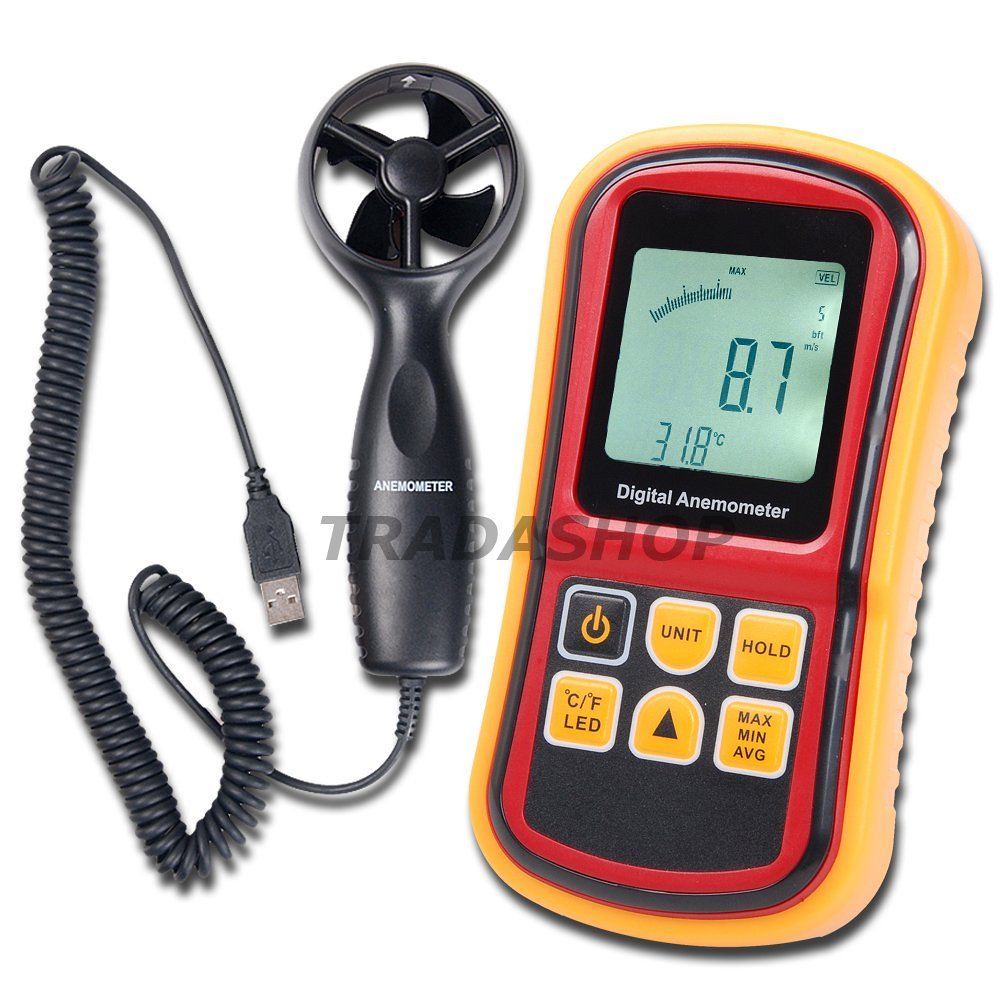The image features a product photo of two distinct yet complementary devices positioned against a white background. The device on the left is black with a coiled, telephone-style USB connector at one end and a fan-shaped design at the other, marked with the word "Anemometer." It is a handheld instrument used to measure wind speed by generating a charge when exposed to airflow. The device on the right is rectangle-shaped with a yellow body, featuring a digital display showing readings like 8.7 and 31.8 degrees Celsius. Below the display, it is labeled "Digital Anemometer" and includes six buttons, each marked for various functions such as power, unit selection, hold, Celsius/Fahrenheit toggle, a right-side-up triangle, and Max/Min/Average. The word "Tradershop" is superimposed in the center of the image as a watermark.